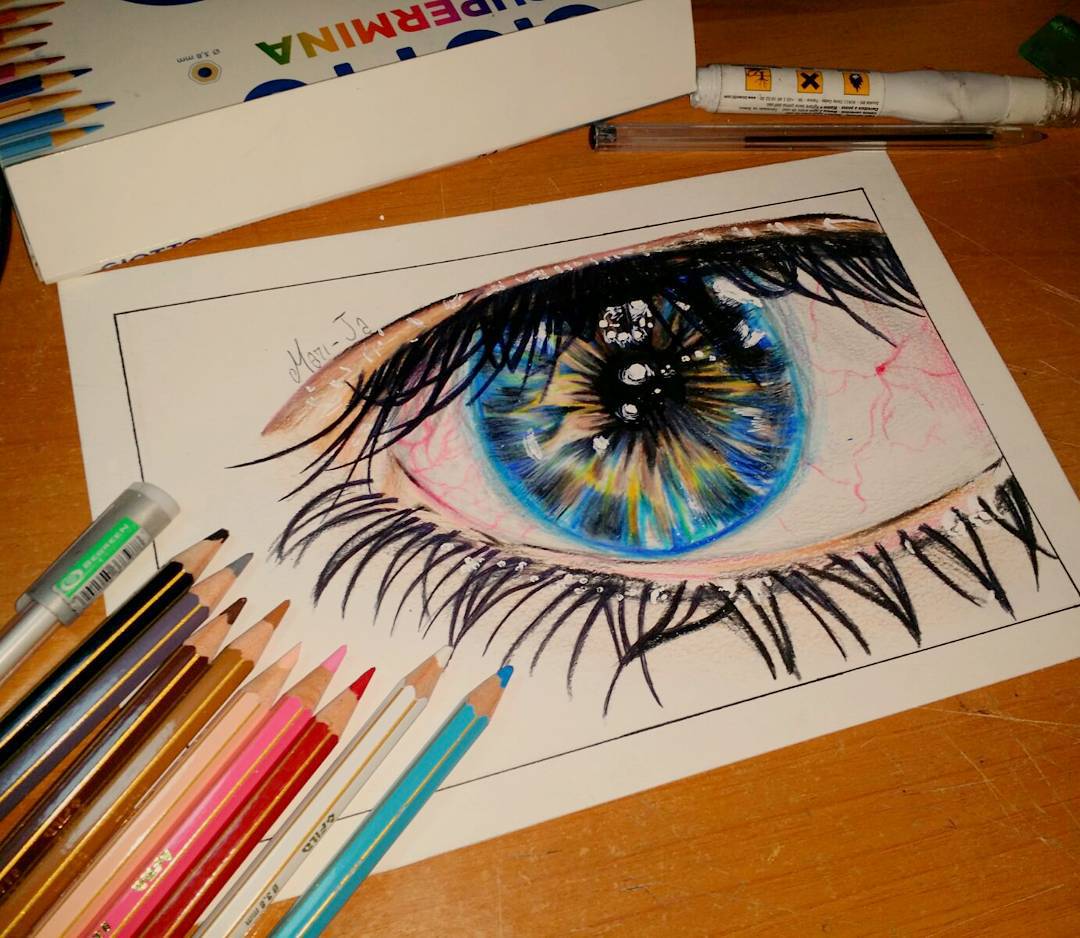The close-up photograph captures an elaborate colored pencil drawing on a white piece of paper, slightly tilted to the left, positioned centrally within the image. Dominating the composition is a highly detailed eye, enveloped by a thin black border. The iris of the eye is a vivid blue, interspersed with striking orange rays, and features a black pupil highlighted with white spots. The eye boasts thick, long black eyelashes and discernible top and bottom lids, shading in hues of peach and brown. Adjacent to the paper, in the lower bottom left corner, lies an array of colored pencils, including shades like light blue, white, red, pink, flesh tone, gold, brown, purple, cyan, dark blue, and black, along with a pen marked by a white and silver lid. These art supplies rest on a light brown wooden table, bearing white scratches on the right side. Additionally, a white rectangular box featuring images of colored pencils and multicolored lettering is partially visible to the left, hinting at the art brand yet obscured. The artist's signature, "MA71-JA," is inscribed on the paper, adding a personal touch to the intricate scene.